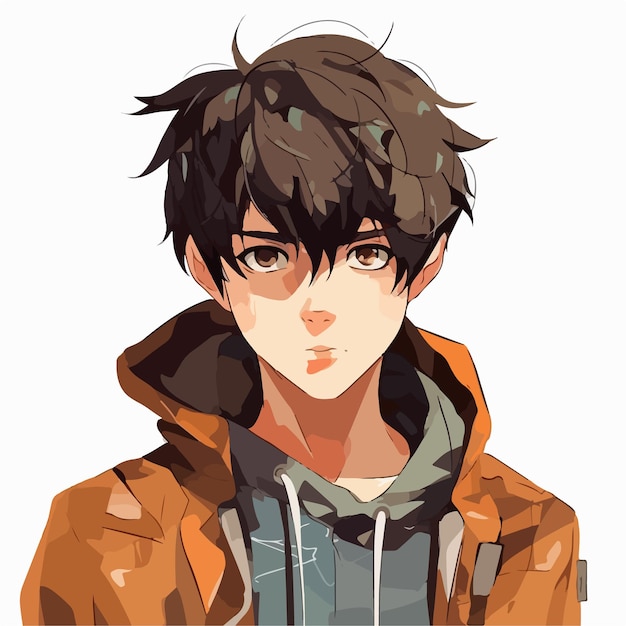The image appears to be a meticulously detailed still from an animated movie or cartoon, featuring a young boy with a neutral expression. The background is predominantly white, providing stark contrast and drawing attention to the character. The boy looks around eight years old, with an oval-shaped face and a pointed chin. His large brown eyes and brown eyebrows stand out, giving his face a touch of lifelikeness, while his petite nose and lips further accentuate his youthful appearance.

He has a distinctive hairstyle, with dark black hair that has a hint of brown at the crown. His hair is somewhat mid-length and messy, with pieces that extend just past his ears and bangs that slightly obscure his forehead and parts of his face, adding to his somewhat disheveled look. 

The boy’s attire is layered, starting with a white T-shirt at the base. Over this, he is wearing a greenish hoodie with white drawstrings, and on top of this, he has a brown camouflaged jacket that features a burnt orange hood. The jacket also includes a gray camouflaged area at the center, and its own drawstrings are visible around the neck area. Both hoods in the layered clothing are down, allowing the viewer to see the ties clearly. The character's pointy ears peek out from his hair, and the shadows and highlights throughout the image enhance the detailed and lifelike appearance of his hair, face, and clothes. His expression leans towards a bland or slightly sad demeanor, further adding depth to his character in this animated still.